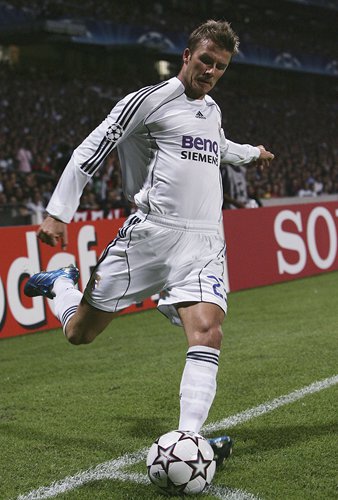The photograph captures soccer star David Beckham in an intense moment mid-strike, preparing to take a corner kick. Beckham, known for his short blonde hair and focused expression, wears a white long-sleeved uniform top featuring the name "Bennis Siemens" along with an illustration of a soccer ball. His outfit includes matching white shorts with a distinctive blue diagonal pattern and black-striped, high white socks. In this dynamic shot, his right leg is pulled back for the kick while his left leg firmly grounds him. His left arm is extended outwards for balance, with his right arm stretched similarly for stability. The soccer ball, marked with a unique star pattern, is poised next to his foot on the green field bordered by white lines. Behind Beckham, a packed stadium is visible, divided from the pitch by a red barrier emblazoned with a Sony logo. The scene suggests a high-energy match, evident from Beckham's sweaty, tousled hair, indicating he has been actively playing for some time.